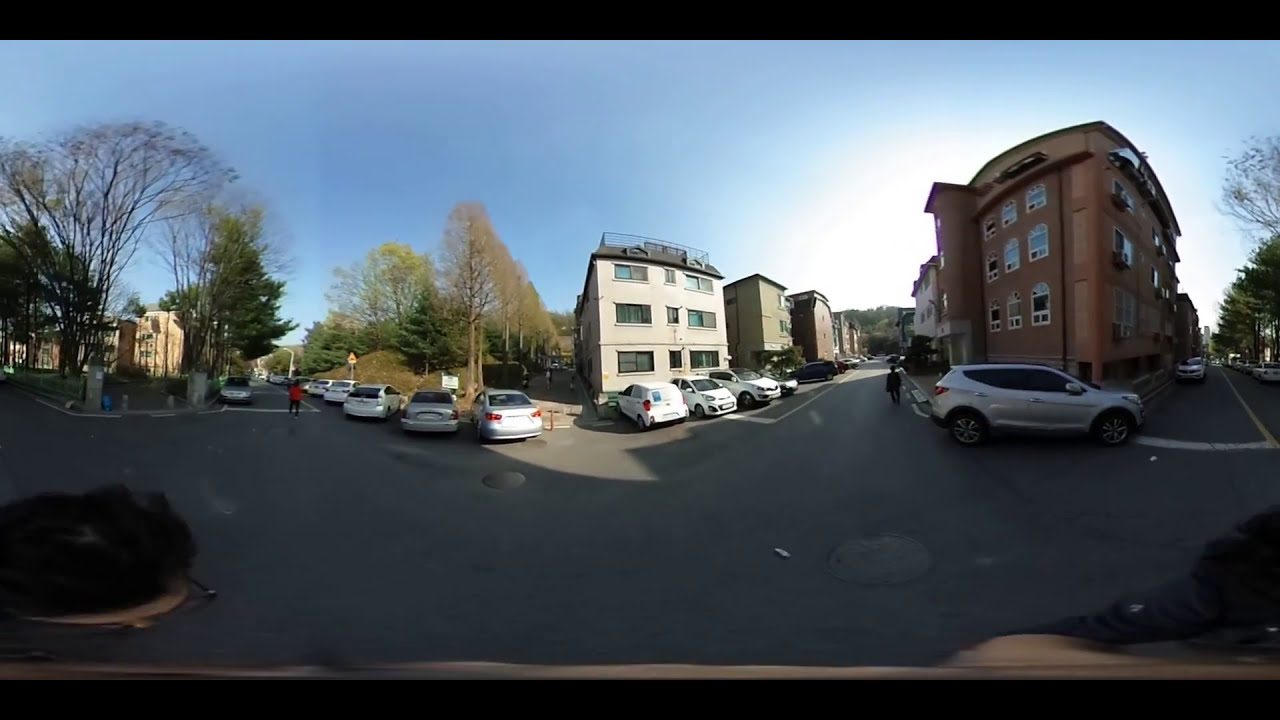The photo depicts an outdoor scene in what appears to be a residential apartment neighborhood, likely in Europe. The shot, captured from a road, possibly by someone on a bike or motorbike, offers a wide-angle view of a parking lot filled with various cars, including white, silver, blue, and red ones. The buildings in the background are predominantly four stories high and showcase a mix of architectural styles and colors: There are white, sandstone-colored, tan, and brick-colored flats. The scene includes a mix of greenery, with trees that have green leaves, some bare branches, and reddish-brown leaves, indicating a transitional season. 

Two individuals can be seen: one walking away from the camera along the road in a red jacket, and another wearing a dark-colored jacket and trousers. There are notable black lines across the top and bottom of the image, possibly an artifact of the camera. Additional details include some green bushes growing out of a brick-lined area on the bottom-left, and white lines on the asphalt indicating road or parking lot markings. The overall setting is a vibrant residential space with a variety of parked cars and people moving about.